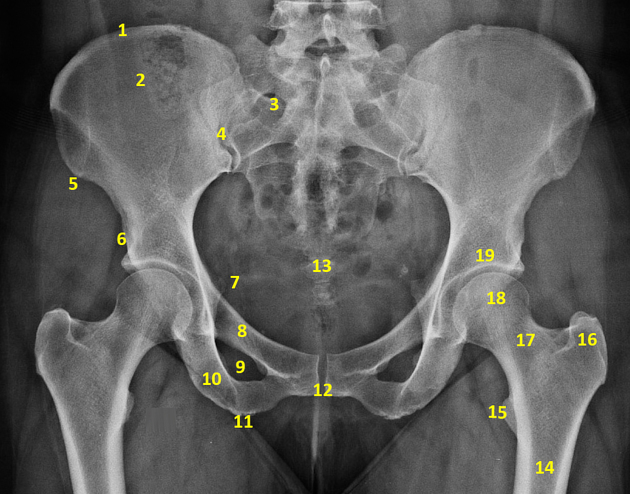The image depicts a detailed black and white x-ray of a human pelvis, showcasing the pelvic bones, spine, hip joints, and the iliac crests with exceptional clarity. The x-ray, presumably educational, features yellow numbers ranging from 1 to 19, each strategically placed on different parts of the skeleton to possibly signify specific anatomical landmarks. Despite the apparent lack of accompanying text to explain the numbers, they stand out distinctly against the black and white backdrop, suggesting the image's use as a reference tool, likely in a medical or educational setting. The health of the bones appears to be normal, with no visible cracks or anomalies. The overall layout, including the pelvic bowl and thigh joints, supports the notion that this is an instructional image designed to aid students, doctors, or nurses in identifying and learning about the various bones within the pelvic region.